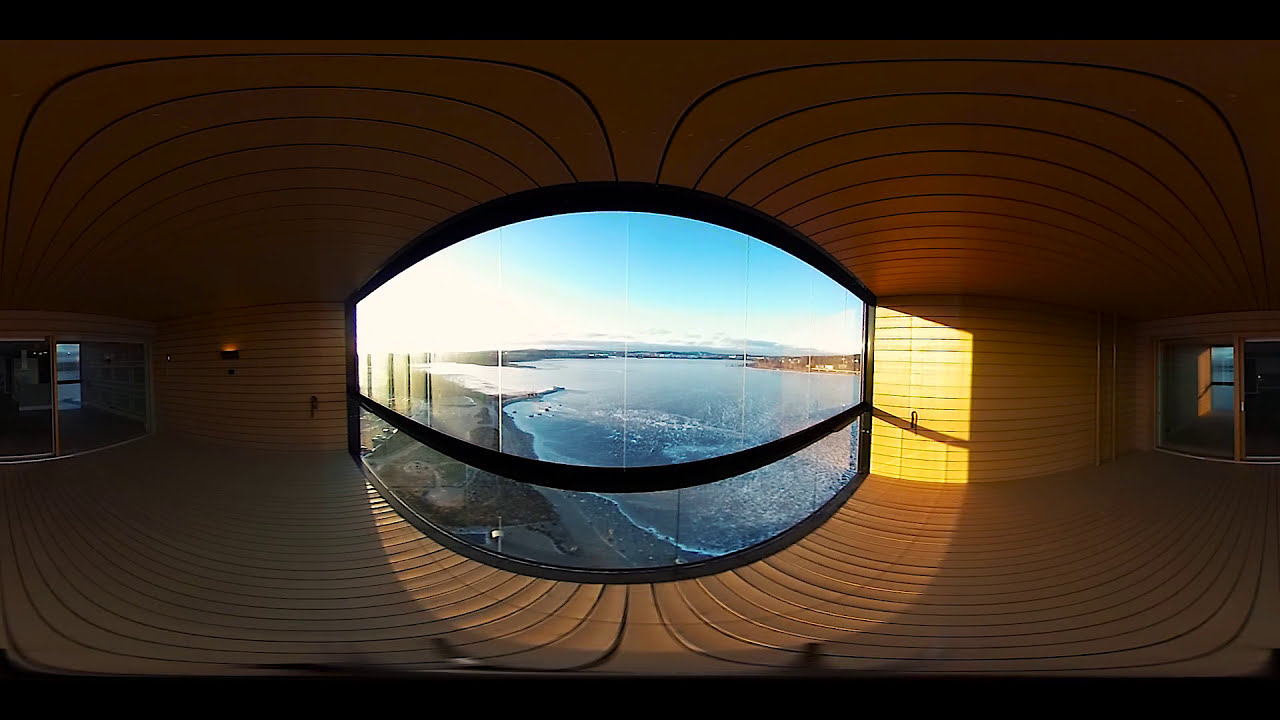The panoramic photograph captures a serene view from the interior of an empty building overlooking a body of water, possibly an ocean or a lake. The interior features wooden floors and walls, with a matching wooden ceiling, creating a cohesive earthy tone that contrasts with the blue water seen outside. The photograph appears slightly warped, indicative of a 360-degree view. A floor-to-ceiling glass window or lucite balcony railing provides an unobstructed view of the calm water gently lapping against the shoreline, with a town visible on the far right and distant mountains. The curvature of the window adds a dynamic element to the scene. Inside, the room is largely bare, save for a doorway to the right, and the space is bathed in natural light creating bright yellow patches on the walls, suggesting a setting sun. The vivid blue sky gradually fades to white towards the horizon, enhancing the tranquil, picturesque quality of the scene.